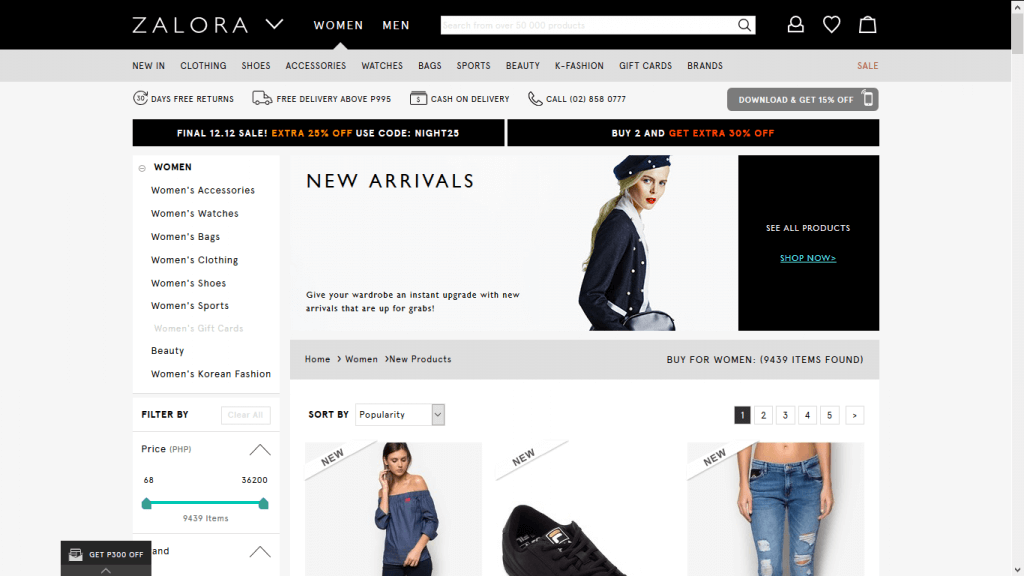The image appears to be a screenshot of the Zalora website. The top portion features a black bar with the Zalora logo prominently displayed. Adjacent to the logo are dropdown menus labeled "Women" and "Men," followed by a search bar. To the right of the search bar are icons for a user account, a favorite items list (heart), and a shopping bag.

Below the top bar is a navigation menu with categories for "New In," "Clothing," "Shoes," "Accessories," "Watches," "Bags," "Sports," "Beauty," "K-Fashion," "Gift Cards," "Brands," and a "Sale" section highlighted in red. 

Beneath the navigation menu, there's a banner showcasing various benefits such as "30-day free returns," "Free delivery above P99.5," and "Cash on delivery." Contact details including a phone number and a promotional message about downloading the app for an additional 10% discount are also featured.

The main content area displays a series of images: a woman wearing a hat and jacket, another woman in an off-the-shoulder blue blouse, a shoe, and a pair of jeans. 

On the left-hand side, additional categories are listed: "Women," "Women's Accessories," "Women's Watches," "Women's Bags," "Women's Clothing," "Women's Shoes," "Women's Sports," "Beauty," and "Women's Korean Fashion." There's also an option to filter items by a specific area, and a "Shop Now" button encouraging users to see all products. Additionally, a price filter allows users to set a maximum price for the items displayed.

This comprehensive layout provides users with diverse navigation options, various product categories, and enticing promotional offers, effectively enhancing the shopping experience on the Zalora website.